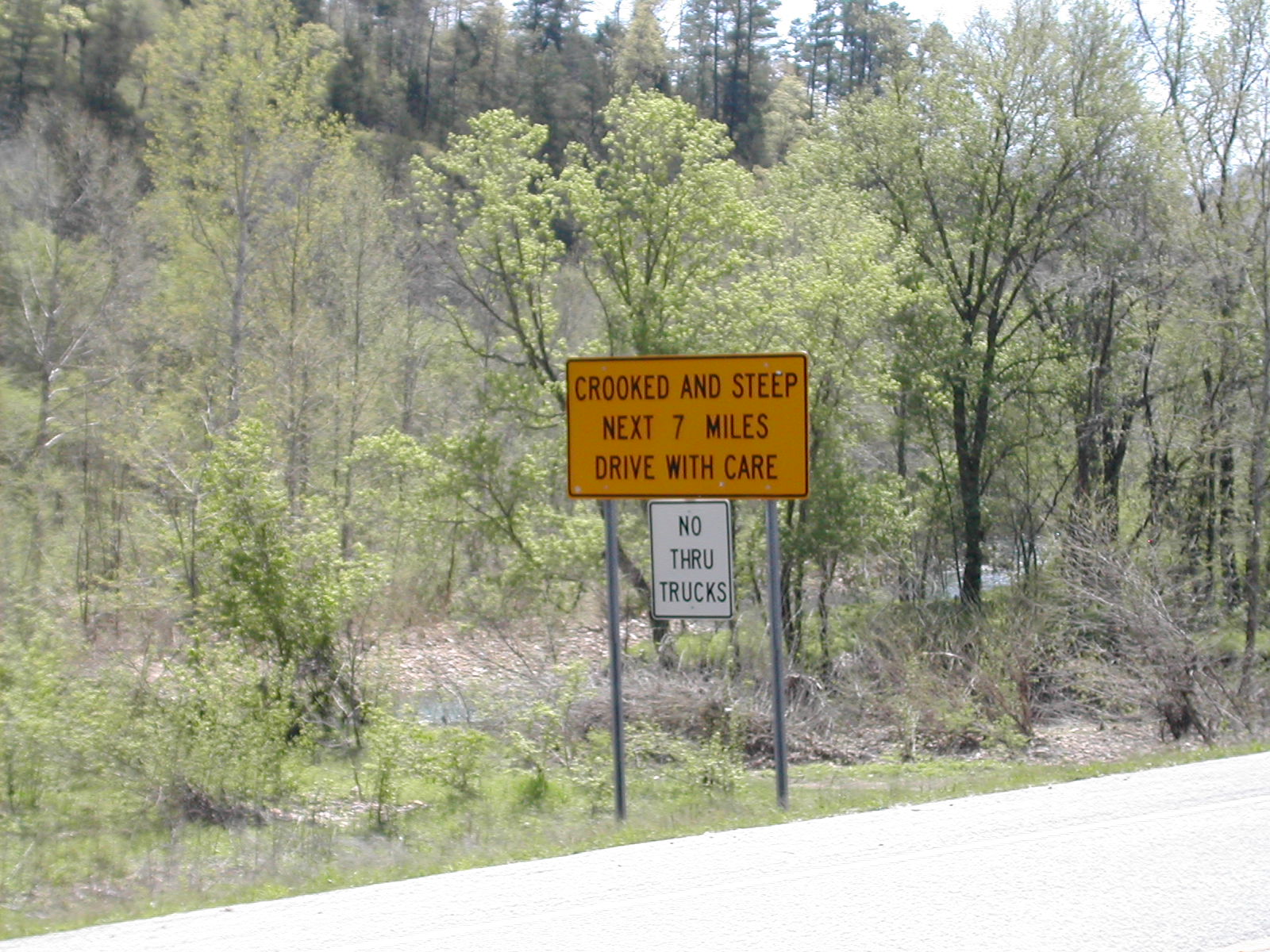In this slanted image, a vivid orange road sign stands prominently in the center, slightly tilted towards the left. The sign warns, "Crooked and Steep, Next 7 Miles, Drive with Care." The photograph appears angled, suggesting that the bottom right corner depicts a gravelly, cement road, which is brightly illuminated, blending with the lighter background. This peculiar perspective gives the entire scene a distinctive, almost tilted appearance.